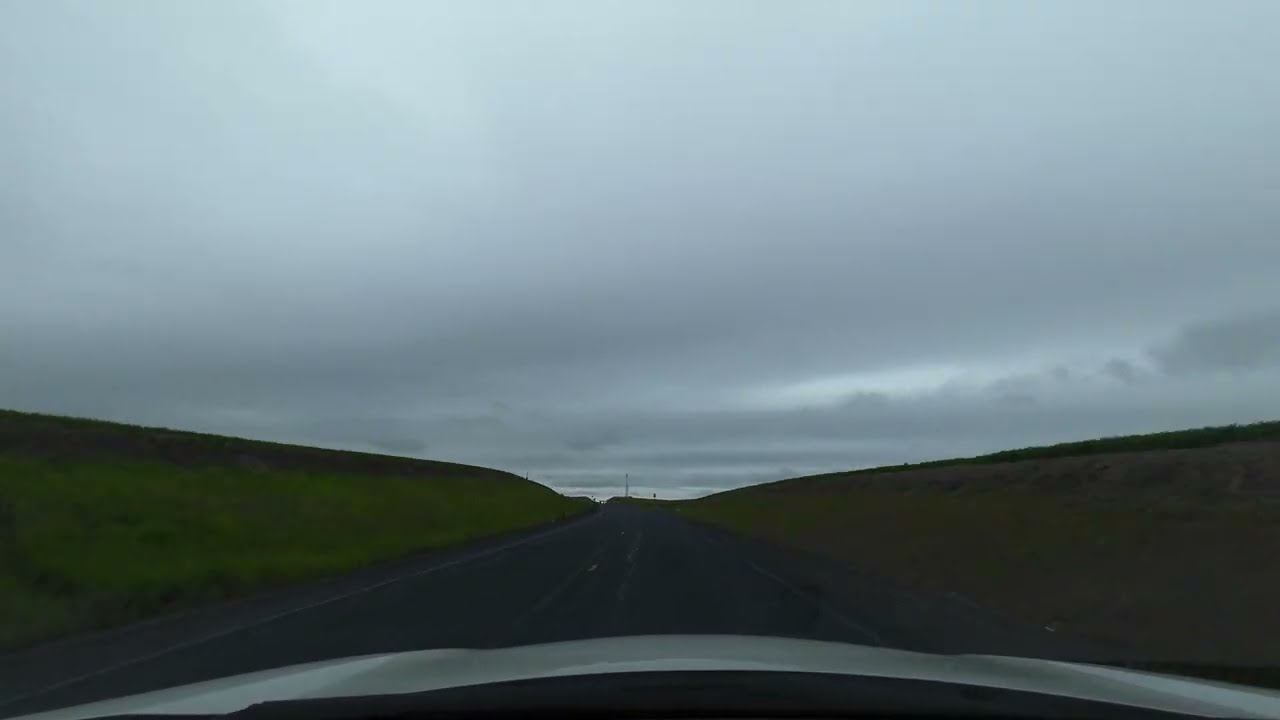The image depicts a road scene captured from inside a car, with the hood of the vehicle—a gleaming silver—visible at the bottom edge of the frame. The car is traveling on a dark asphalt road marked with faint white lines. The scene extends straight down the road, flanked by raised hills on either side. On the left, the hill features vibrant green grass transitioning to a darker brown towards the top, while the right side showcases primarily brown terrain with patches of darker green, likely indicating trees, as it meets the horizon. In the far distance, vertical structures such as power lines or towers can be discerned against a heavily overcast sky. The sky is dominated by thick, gray stratus clouds, giving the impression of an impending rain and casting a dim, somber light across the landscape. The overall atmosphere is dark and somewhat foreboding, accentuated by the heavily clouded, whitish-gray sky that obscures any hint of sunlight.